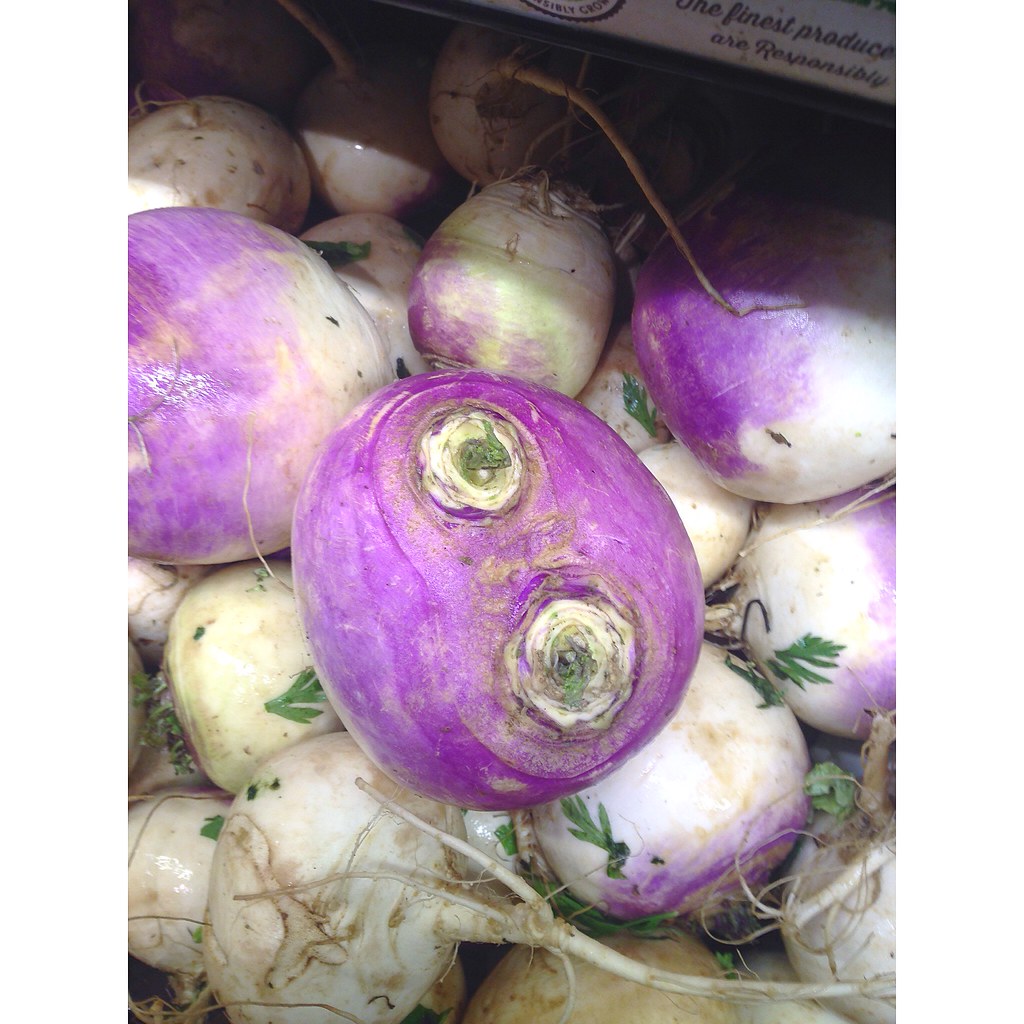This image captures a heap of vegetables that resemble onions, turnips, or possibly parsnips, piled together in a disorganized manner inside a bin or crate. The majority of these vegetables are white, but many display patches or layers of purple skin. Some of them have attached green leaves, suggesting they were freshly dug up. The vegetables appear moist, likely from being misted. A few of them show long, untrimmed roots. In the upper right-hand corner of the image, there's a partially visible sign that reads “finest produce” and mentions something about being “responsibly grown.” This scene likely depicts a collection of purple-tinged root vegetables, possibly stored for sale at a marketplace or a supermarket.